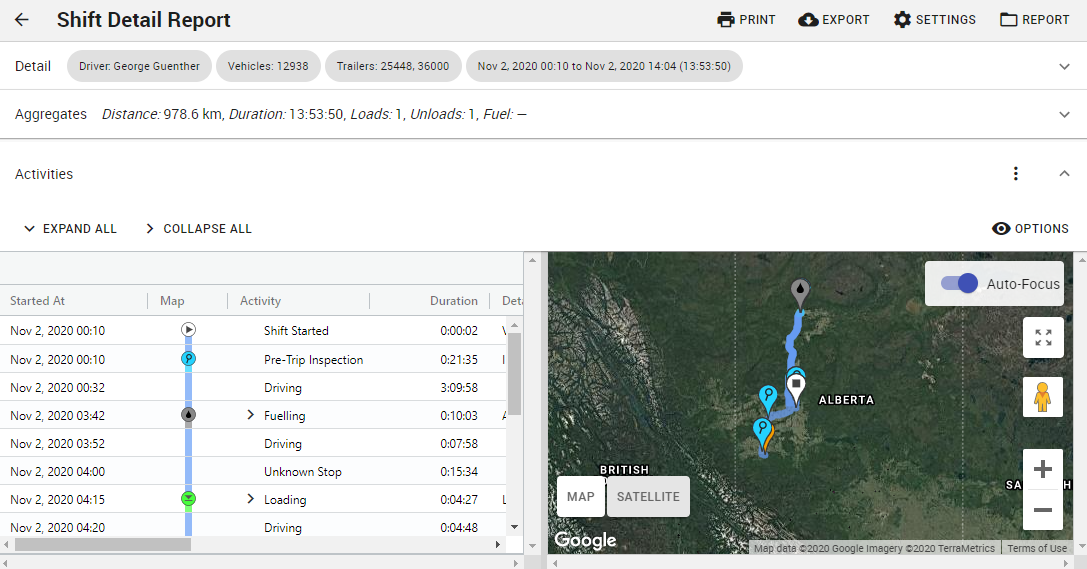In the top left corner of the image, there is a "Shift Detail Report." The top section of the document highlights various settings, such as print and export options. It provides a detailed report for the driver, George Grunter, who operates vehicle number 12,938 and trailer number 25,448, with a combat identifier of 36,000. 

The report covers activities from November 2, 2020, to November 2, 2022, at 2:00 PM, detailing an aggregate distance of 978.6 kilometers covered over a duration of 13 hours, 53 minutes, and 50 seconds. It records one load and one unload event. The fuel activities section includes options to expand or collapse details and started map activity duration columns.

Additionally, the map in the image shows several locations, including British Columbia and Alberta. Smaller text on the map indicates "Map data copyright 2020 Google" and "Imagery copyright 2020 Diametrics," adding context to the visual data presented.